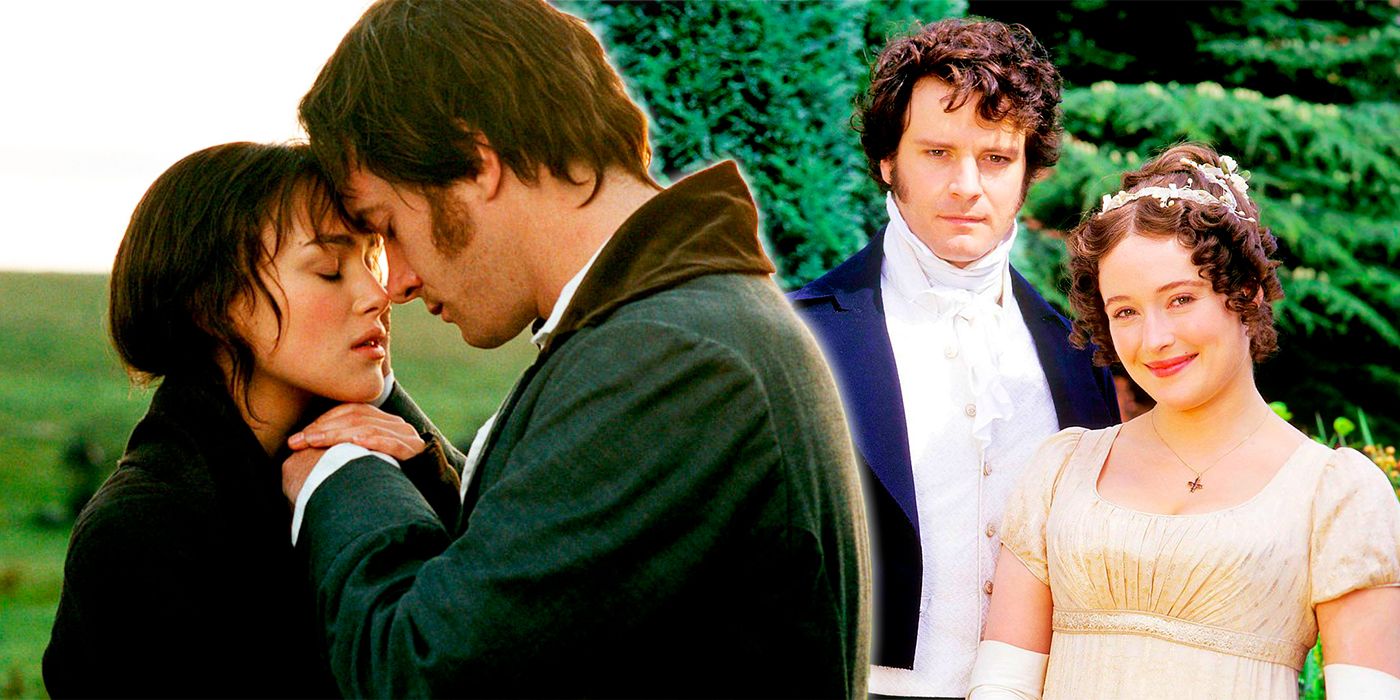This image is a collage of two distinct scenes reminiscent of a romantic period drama, possibly from the movie "Pride and Prejudice." On the left, we see a highly intimate moment featuring a man and a woman, likely Keira Knightley and a male co-star, in a close embrace. Their foreheads touch and their eyes are closed, conveying a deep emotional connection. The man, sporting prominent sideburns, wears a dark green jacket over a white undershirt, and gently cradles the woman's face with his right hand while holding her hand below her chin with the other. The woman dons a dark black coat. This tender scene is set against a backdrop of grassy fields under a clear sky.

On the right side, another couple stands in formal Victorian attire, suggestive of a different thematic scene. The man, with a stern and intense gaze, is dressed in a blue fancy suit coat over a white button-down shirt, accessorized with a white ascot. Beside him is a woman in a yellow gown, smiling warmly with flowers adorning her hair. The background features lush greenery, including trees and bushes, further emphasizing the period piece setting. Both scenes together create a vivid portrayal of romance and elegance in a bygone era.